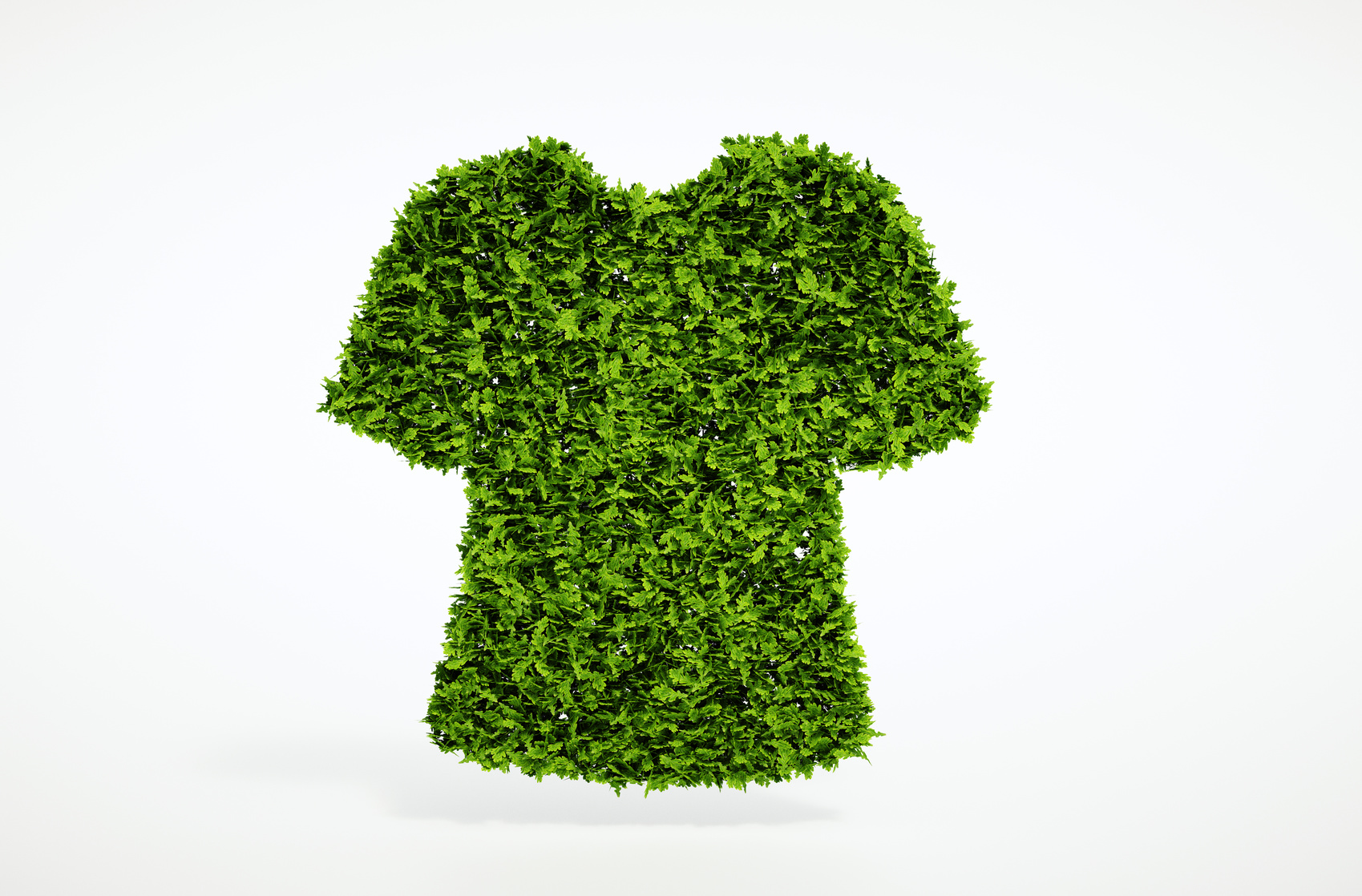This image is a detailed digital artwork featuring a unique depiction of a t-shirt crafted entirely from green leaves. The shirt appears to be made from finely detailed, dark green foliage that transitions to lighter green at the edges, showcasing a delicate frilled texture with small white gaps peeking through. The leaves are densely packed, creating a clear and distinct t-shirt shape with short sleeves and a slight U-neck. The rectangular image, approximately six inches wide by four inches high, has a faint light blue background that transitions to light gray at the corners. A subtle gray shadow beneath the leafy shirt suggests it is floating slightly above the background, adding a touch of depth to the piece.